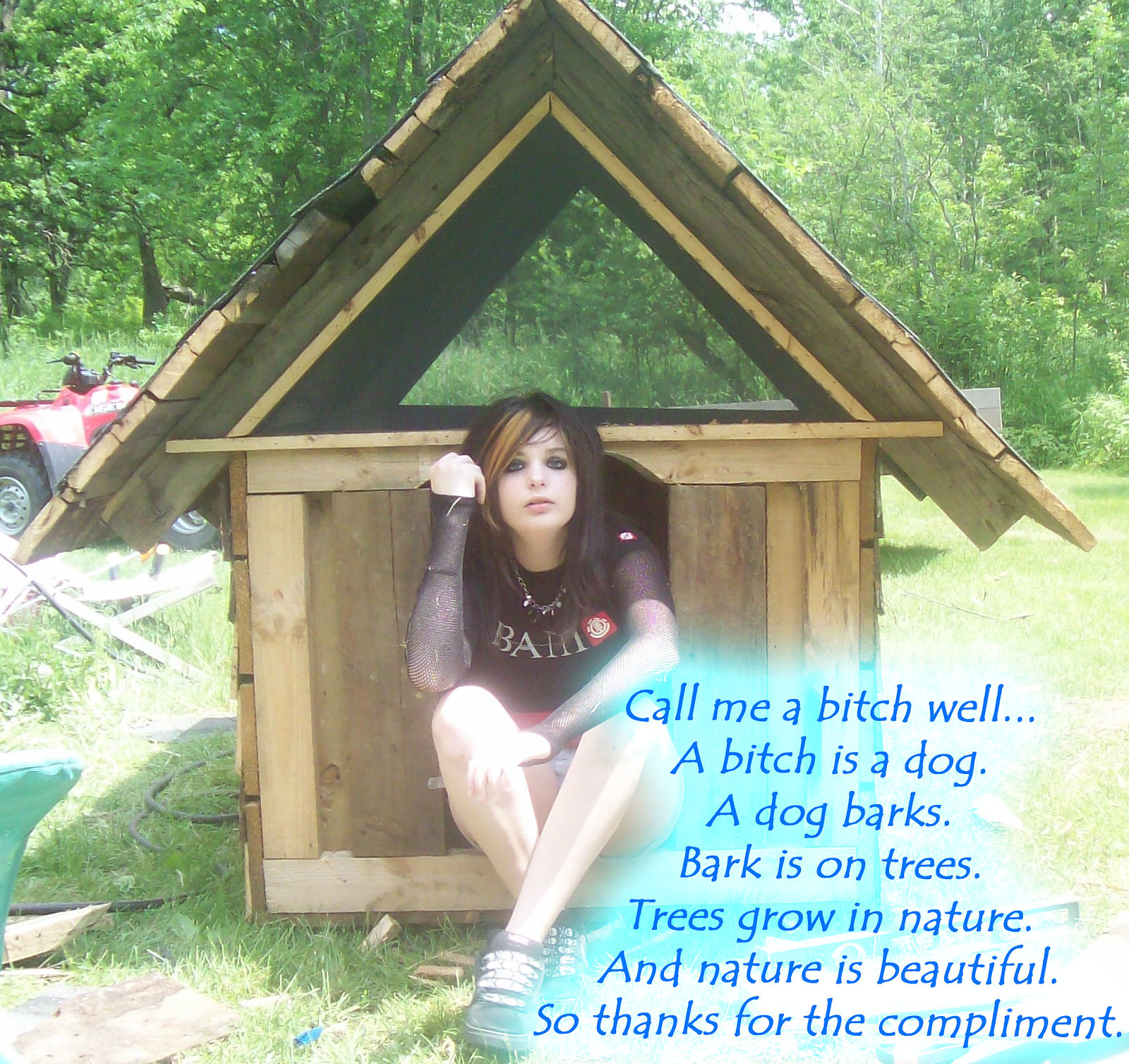The image features a teenage girl, approximately 15 or 16 years old, with a goth or emo style. She has medium-length black hair accented with a streak of blonde or purple. The girl is sitting at the entrance of a wooden doghouse, with her bottom just inside the small structure. Dressed in a black sheer shirt with a design that might say "bath" or "bam," she also wears mesh sleeves that extend to her hands, along with shorts and black sneakers. Her striking makeup includes heavy black eyeliner and possibly eye shadow. Surrounding her, there is lush green grass and trees in the background, adding to the natural ambience of the scene. In front of her, a blue-text caption with a light blue halo effect reads: "Call me a bitch. Well, a bitch is a dog. A dog barks. Bark is on trees. Trees grow in nature, and nature is beautiful. So thanks for the compliment." An ATV can also be seen off to the side, and the girl gazes directly at the camera with a calm demeanor.